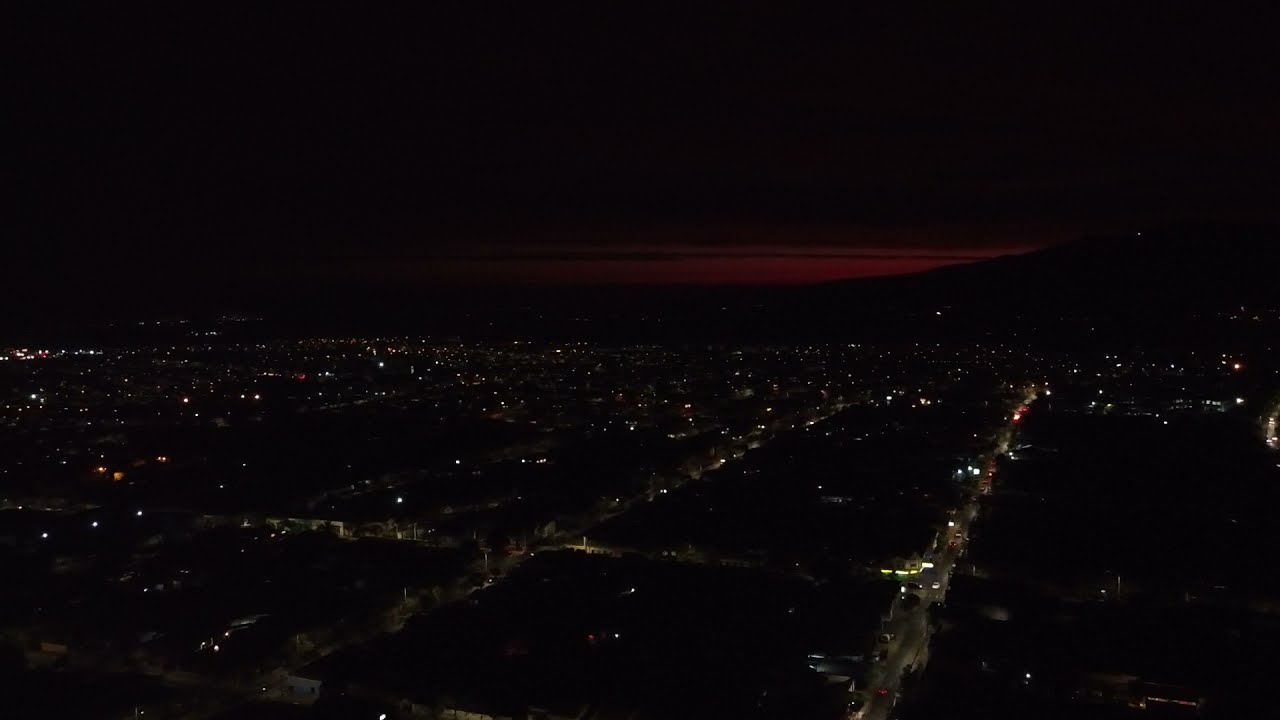This nighttime aerial photograph captures a sprawling cityscape, possibly taken from a higher vantage point such as a hill or an airplane. The city is illuminated with numerous lights that resemble stars scattered across the ground due to the distant viewpoint. The lights trace a grid-like pattern indicative of road networks, with a notable road extending across the scene, dotted with moving vehicles.

In the foreground, the city appears to consist mostly of one- and two-story buildings, suggesting a small town rather than a metropolitan area. The sky above is predominantly dark, signifying the late hour, but there's a striking expanse of reddish-orange streaks on the horizon, hinting at a recent sunset. These warm hues gradually transition to a deep brown and then to the blackness of night.

In the distance, the silhouette of a mountain or hillside slopes gently across the horizon, adding depth to the landscape. Overall, this image beautifully juxtaposes the intricate, illuminated layout of the city against the serene, fading colors of a twilight sky.